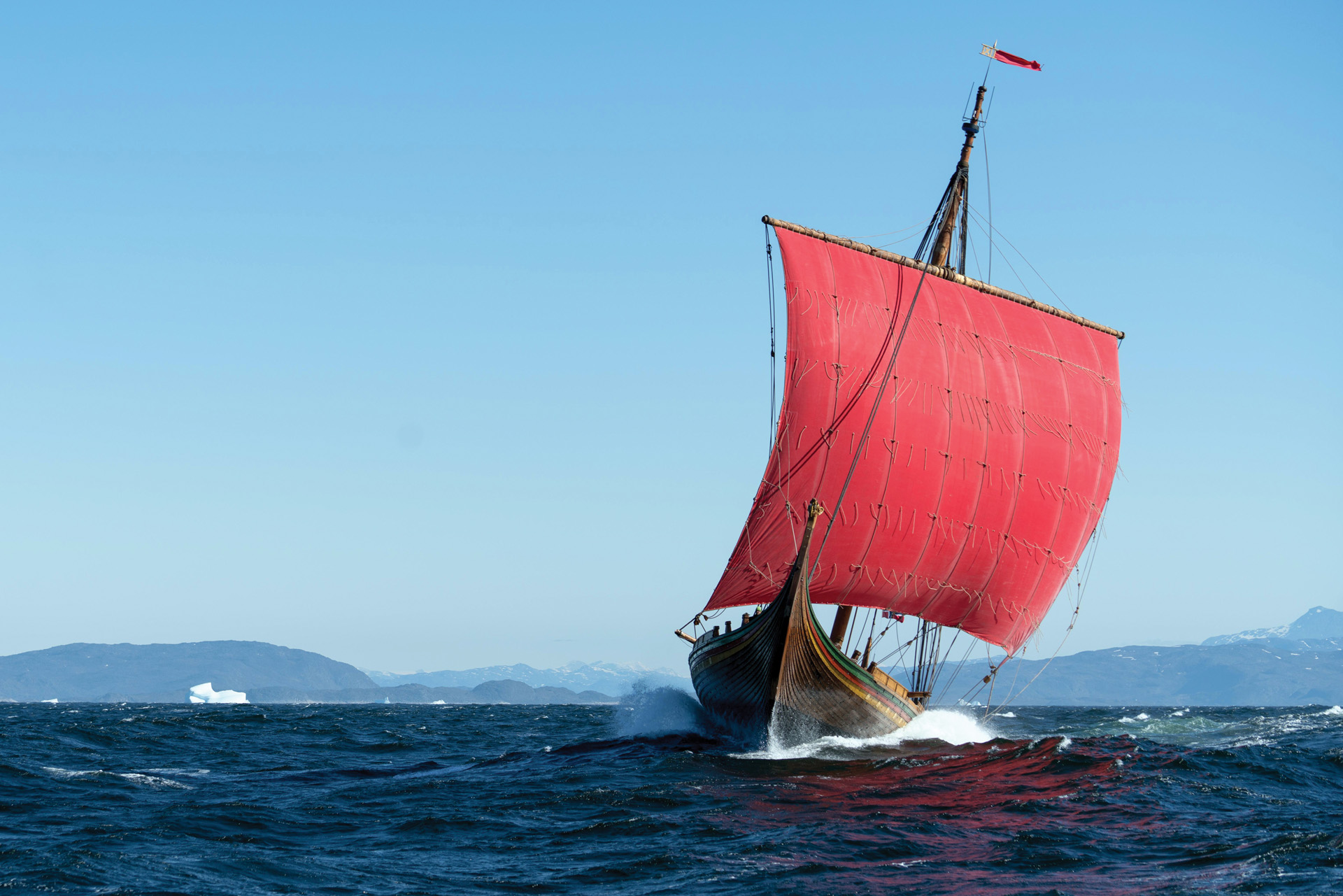In this captivating ocean photograph, the viewer is presented with a striking maritime scene set against a backdrop of distant hills and a serene shoreline. Dominating the foreground is a solitary, majestic sailboat with a distinctly vintage design reminiscent of a Viking ship. This wooden vessel, polished to a dark black at the hull and transitioning to a rich brown towards the top, features intricate stripes of yellow, red, and green just beneath its edge.

The boat is steered by a single, expansive square sail that is a vivid red, puffed out fully by the forceful wind propelling the vessel. At the top of the center mast, a slim red flag flutters briskly. Amidst the calm, low waves of the deep blue ocean, the sailboat surges forward, the waves splashing on either side with palpable energy.

The sky overhead is a clear, unblemished blue, adding to the tranquil yet vibrant atmosphere of the scene. In the distant background, a mountain ridge outlines the horizon, adding depth to the landscape. To the far left on the horizon, one can spot a futuristic, curvy white building, adding an unexpected modern touch to the otherwise timeless maritime voyage. The photograph is devoid of any additional ships or people, keeping the focus solely on the impressive sailboat and its dynamic interaction with the ocean.